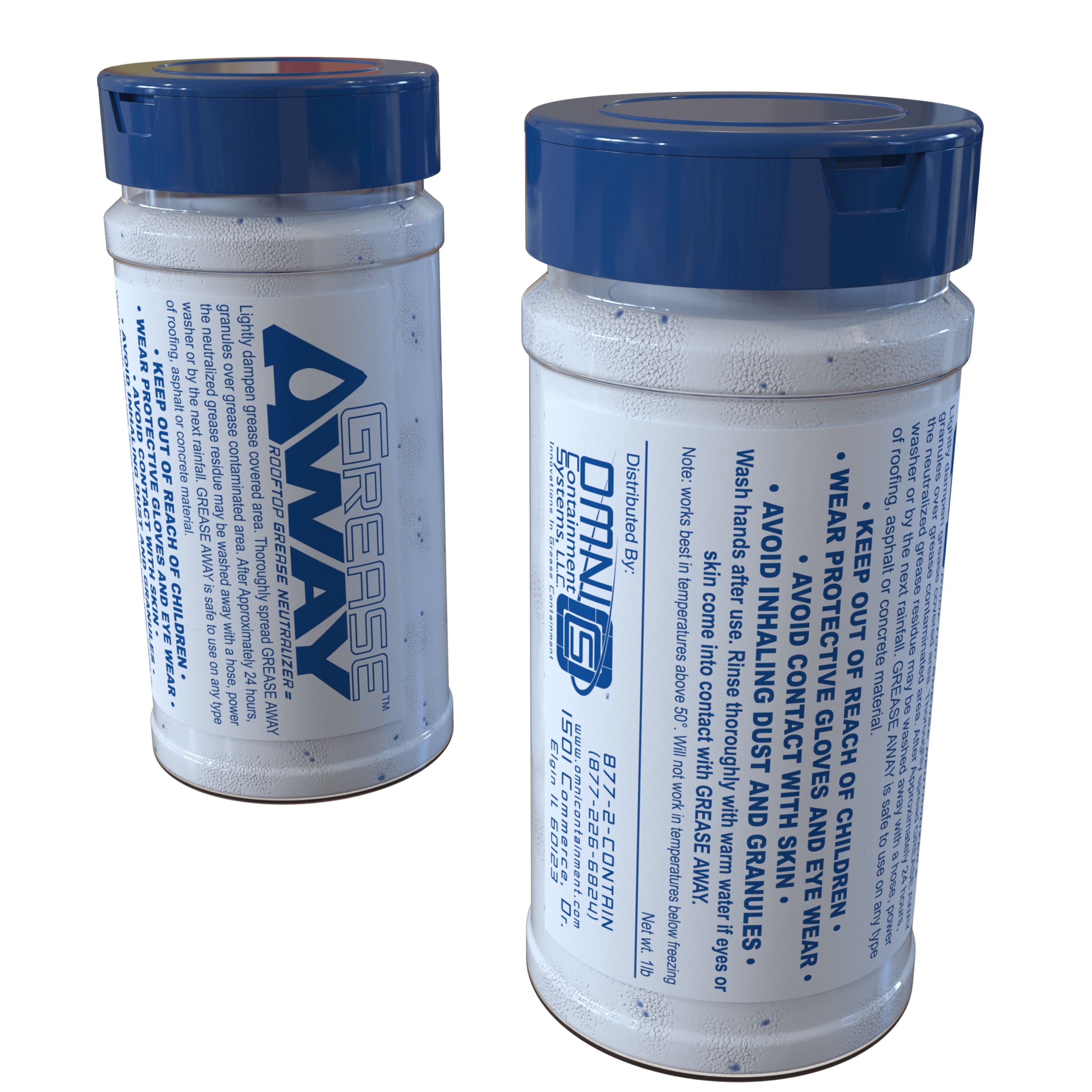The image depicts two nearly identical plastic bottles with blue pop-top lids, positioned against a completely white background. The bottle on the left showcases the front label in blue and white text, reading "Grease Away™ Rooftop Grease Neutralizer." Several warning labels occupy the space below, including instructions about keeping the product out of reach of children, and the necessity of wearing protective gloves and eyewear to avoid skin contact. The label also provides usage directions: "Lightly dampen grease-covered area, then thoroughly spread Grease Away granules over the grease-contaminated area." The white powdery substance inside the transparent bottles, speckled with small blue granules, is intended to neutralize grease on various rooftop materials like asphalt and concrete. The bottle on the right reveals the rear view, detailing ingredients and reiterating safety precautions and application instructions, emphasizing its industrial use and inedibility despite the bottle's resemblance to a spice jar.